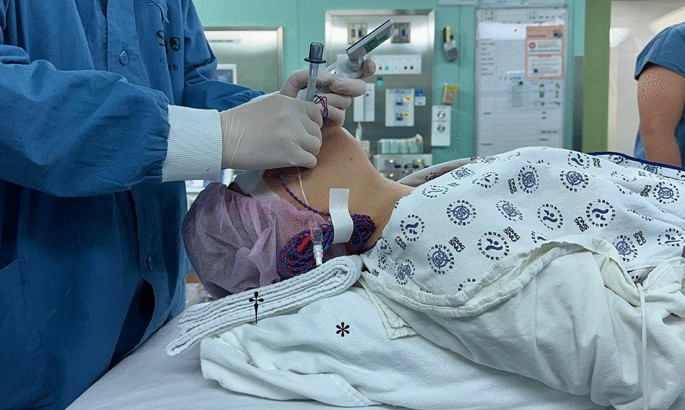In the image, a woman is undergoing a medical procedure in a hospital operating room. She lies on a surgical bed, covered with white sheets and dressed in a hospital gown. Her hair is tucked under a disposable purple cap. Positioned toward the left side of the frame, a doctor in medium blue scrubs with white cuffs and rubber gloves is intubating her, inserting a tube down her throat. Details such as the tape covering her eyes and a towel tucked under her neck are also evident. Surrounding her are various pieces of medical equipment including vials held by the doctor and additional apparatus visible on the teal-colored walls. A whiteboard with handwriting adorns the background, and the partial arm of another medical professional in blue scrubs can be seen on the right side of the image, indicating a collaborative medical environment.